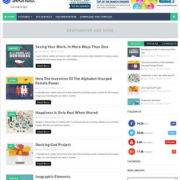This image displays a blurred webpage with a predominantly white background. The central content is arranged in a list format, featuring black text accompanied by images on the left side of each text line. The layout shows two main content columns: one on the left and one on the right. Along the right side of the page, there are three buttons—one green and two navy.

At the bottom right corner, social media icons are visible, including a blue Facebook icon, a light blue Twitter icon, an email icon, and a Reddit icon. On the left side of the page, additional text can be seen alongside black buttons with white text.

At the top of the page, there are navigation tabs—six in total. The first tab is highlighted in green, while the remaining five tabs are navy with white text. In the top-right corner of the image, there are balloons in various colors: pink, green, yellow, and blue.